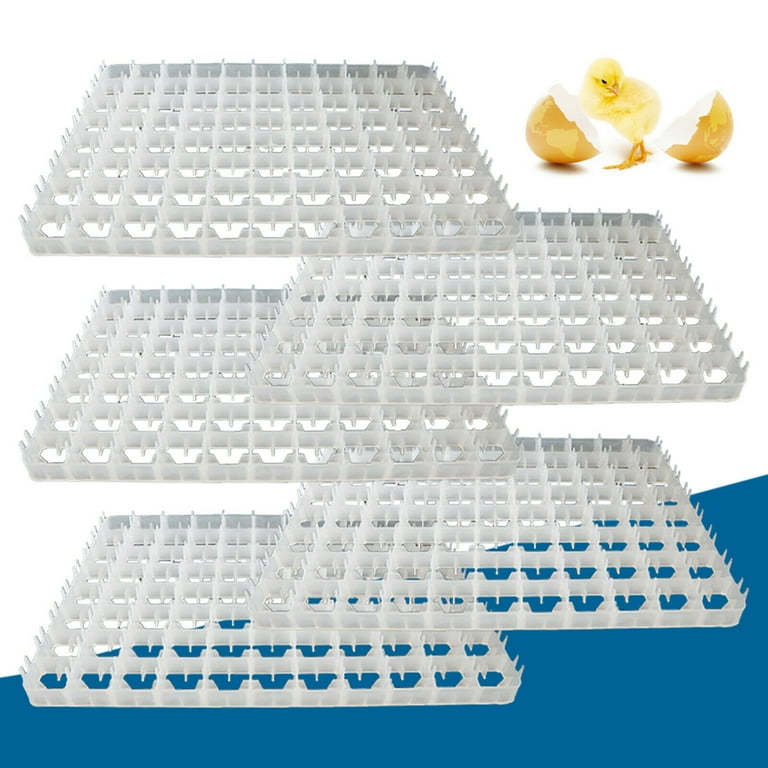This image portrays a highly detailed poster, potentially a brochure page, featuring prominently white, flat, commercial-grade egg crates designed to hold a significant quantity of eggs. Arranged in five large trays, each tray consists of 12 rows, with each row capable of holding a dozen eggs, amounting to substantial storage capacity. Dominating the upper right-hand corner of the image is a charming yellow chick, freshly hatched, flanked by two pieces of its broken eggshell. The chick boasts light yellow fluff and dark yellow feet, adding a touch of life and warmth to the graphic. The background of the image is divided, with the upper portion showcasing a transparent white hue that transitions into a blue stripe at the bottom. The overall design and elements suggest a graphic one might find in farm supply advertisements or online retail platforms, emphasizing the utility and capability of the egg crates in hatching processes or egg storage.